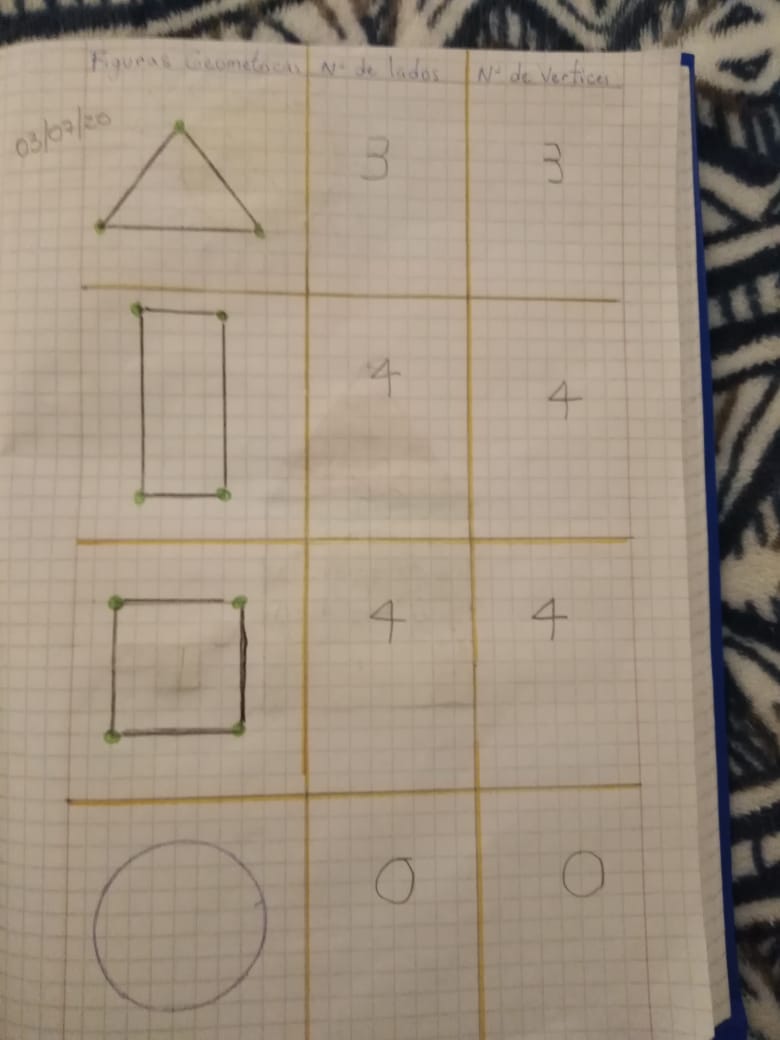This image features a meticulously organized homework assignment displayed on graph paper, which provides a grid-like structure ideal for detailed plotting. The date "03-07-20" is inscribed in the upper left corner, anchoring the temporal context of the assignment. Below the date lies a neatly drawn grid composed of 4 rows and 3 columns, each cell containing specific elements meant for classification or computation. 

In the first row, from left to right, there appears a triangle followed by two occurrences of the number 3. 

The second row showcases a rectangle. Each quadrant of this rectangle is filled with the number 4, suggesting a possible symmetrical division or a calculation exercise within the geometric shape. 

The third row contains a square, similarly divided and populated with the number 4s in its quadrants, maintaining the numerical consistency seen in the rectangle above.

In the fourth and final row, there is a perfectly drawn circle, with its quadrants each containing the number 0, indicating a different computational or categorical approach compared to the previous shapes. 

At the very top of the grid, there is a header written in Spanish, presumably labeling or categorizing the various shapes and numbers presented in the assignment. 

The overall presentation suggests a structured mathematical or geometrical exercise, enhanced by the descriptive labels and precise numeric input, all conveyed within the confines of graph paper to maintain clarity and order.